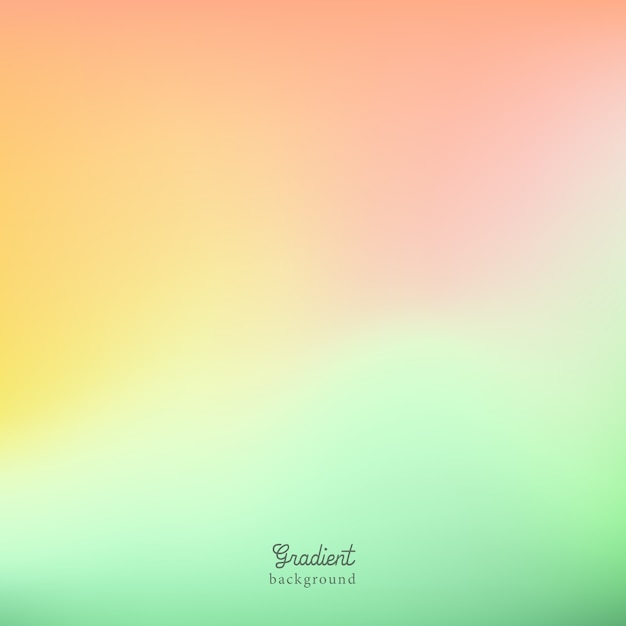The image features a square design with a gradient background split into three distinct colors that intermingle towards the center. The bottom one-third of the image is predominantly green, which gradually lightens and transitions into white as it moves upward. This central white blending area seamlessly merges with the top one-third of the image, which is divided into two sections: the left side has an orange-yellow gradient that becomes more pronounced as it moves rightward, while the right side transitions from orange into a pinkish-red hue. Overlaying this vibrant gradient background in the bottom center are two lines of black text: the top line is a cursive word "gradient," and the bottom line is a straightforward word "background." The overall composition suggests a multi-colored design, possibly the back of a greeting card, distinguished by its smooth color transitions and lack of distinct objects.